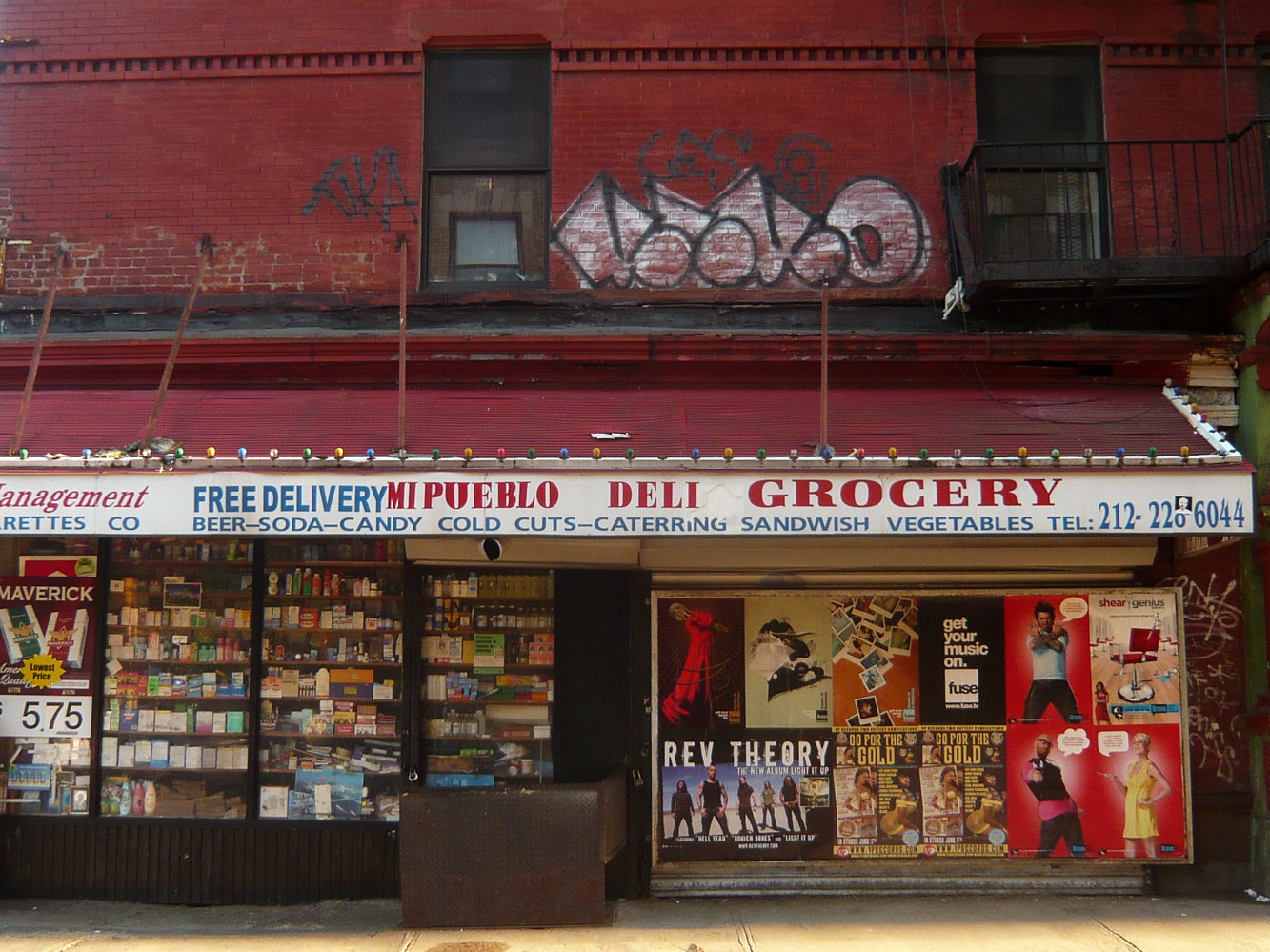In this photograph, we see a red brick building situated on the side of a street. The building features two windows with a fire escape attached to the right window. Above the awning of the store, there is faded graffiti written in white and outlined in black, along with other black graffiti markings. 

The red awning has a white front face displaying various promotional texts: "Management Call, Free Delivery, Mi Pueblo Deli Grocery, Beer, Soda, Candy, Cold Cuts, Catering, Sandwich, Vegetables," followed by the telephone number "212-228-6044." 

Through the store's window on the left, several items, including cigarette displays, are visible. Prominently displayed is a Maverick cigarettes poster with a price of $5.75. On the right side of the window, there are several colorful posters and advertisements, including one promoting listening to music on Fuse and another for Rev Theory.